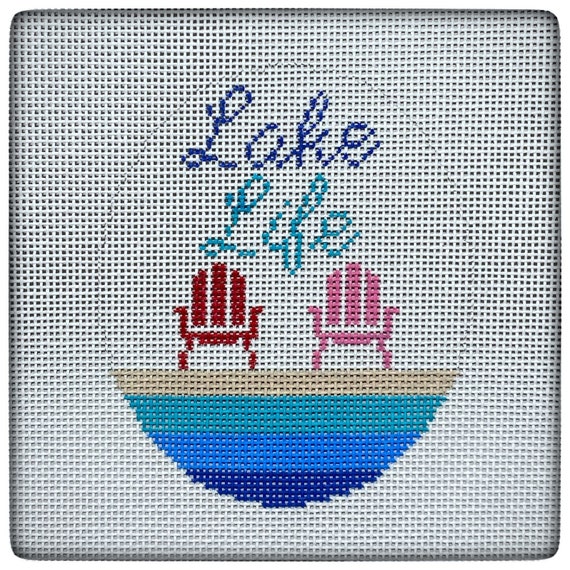A detailed front-facing view of a meticulously hand-stitched, square-shaped mat or coaster made of white mesh fabric with tiny interlocking threads. The center features an oval, enclosing the words "Lake Life" written in cursive, with "Lake" embroidered in dark blue and "Life" in light blue. Just below the text, two wooden beach chairs, the left one burgundy and the right pink, are positioned back-facing towards the viewer. These chairs rest on a sandy-colored strip, representing a beach. Beneath the sand, a gradient of ocean water is depicted with three distinct bars: light blue, blue, and dark blue, beautifully capturing the transition of water depths. This piece, perhaps intended for indoor use, showcases the intricate texture and craftsmanship of the fabric.